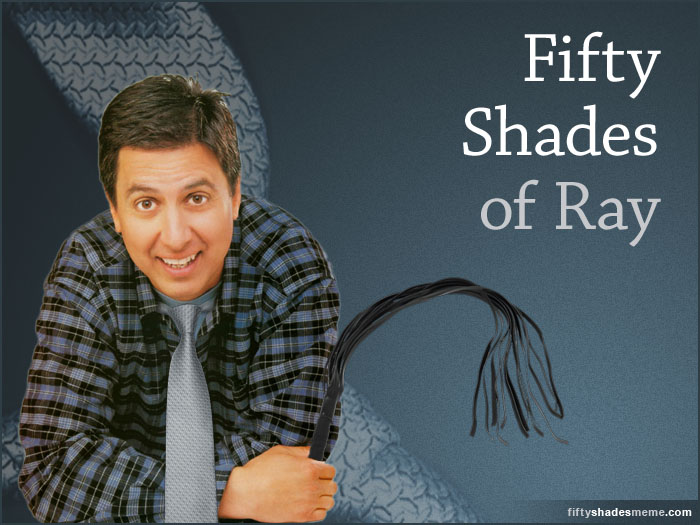The poster image advertises "50 Shades of Ray" with the text displayed in large white and light gray font at the top right. In the bottom right corner, the site "50shadesmeme.com" is written in alternating gray and white font. The left side of the poster features a smiling, middle-aged man with short brown hair, dressed in a blue and black checkered shirt and a light blue tie. He is leaning on his elbows and holding a black whip in one hand. The background is a dark blue-gray shade, with a white tie prominently displayed behind the man.